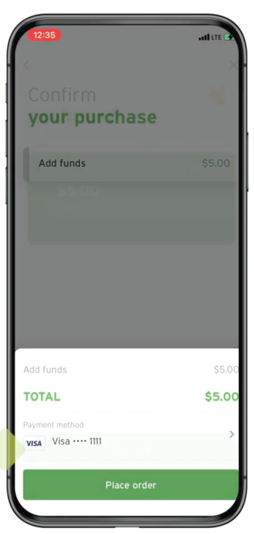This image, captured from a cell phone, shows a screenshot of a transaction page. At the top, the time is displayed in red as 12:35. On the right side, the battery icon indicates it's charging, highlighted in green with black bars inside the battery icon, alongside the LTE signal indicator.

Midway down, there's a prompt to confirm a purchase. The text "Confirm your purchase" is divided, with "Confirm" in gray and "your purchase" in green. Beneath this, there's an option labeled "Add funds," indicating a $5 amount. The lower portion of the screen is blurred, making details obscure, but it’s visible that the grayish upper section contrasts with the more detailed bottom part.

Further down, the total amount is listed as $5 in green. The payment method section shows "Visa" followed by the partial card number "****1111". At the very bottom, a green button extends from left to right with the text "Place Order" boldly written in white.

The screenshot captures a moment on a mobile device during an online transaction, detailing the essential steps of confirming a purchase and specifying the payment method.